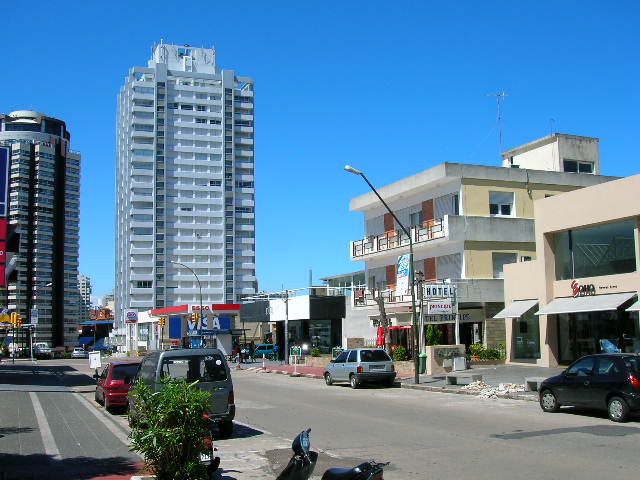The image captures a vibrant cityscape on a bright sunny day with a clear blue sky. Prominently featured are two towering skyscrapers in the background—one circular with numerous balconies and windows, and the other more square-shaped and slightly taller. In front of these skyscrapers, to the right, stands an older three-story yellow building with a balcony and a sign that says "hotel," evoking an old-timey charm.

The street below is lined with several parked cars including black, blue, red, and gray vehicles, suggesting a one-way street as they are parked on both sides. There is no visible pedestrian activity, adding a serene ambiance to the scene. Additionally, a small SO gas station with a red canopy is situated beneath the square skyscraper. In the middle distance, an advertisement for Visa in dark blue with white font is visible, adding a commercial touch to the city setting. The image is predominately concrete, punctuated by a green bush in the middle of the road, completing this bustling, yet tranquil urban landscape.